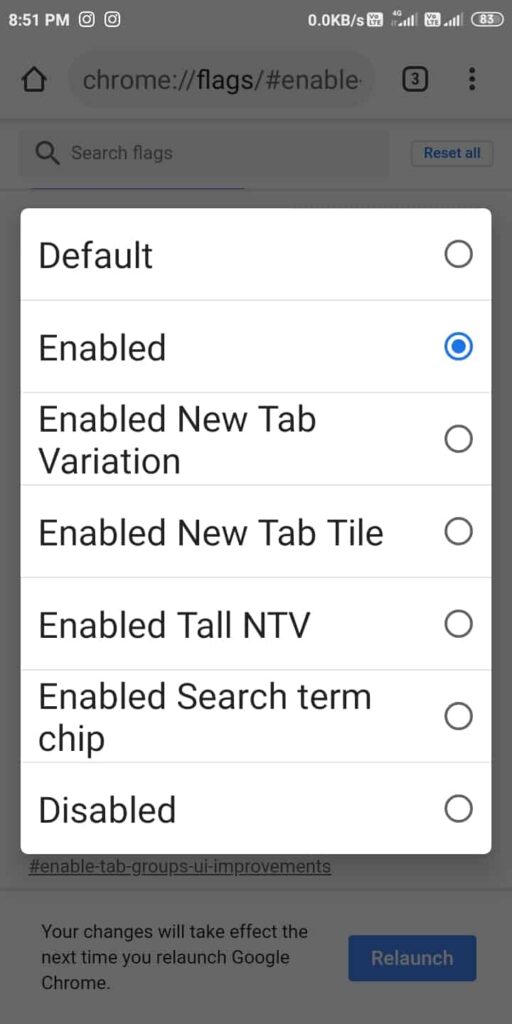This screenshot captures the details of a smartphone display in dark mode or night mode at 8:51 PM, as indicated by the white text in the upper left corner. In the upper right corner, several icons are visible: the LTE signal icon showing 4 out of 5 bars, and the battery icon showing 85% charge remaining. 

Beneath these icons, a Chrome browser address bar displays the URL "chrome://flags/#enable." Directly below the address bar, there is a search bar with the text "Search flags."

The main content of the screenshot is a white dialog box containing various settings. From top to bottom, it reads:

- "Default"
- "Enabled" to which a blue circle is next.
- "Enabled New Tab Variation"
- "Enabled New Tab Tile"
- "Enabled Tall and TV"
- "Enabled Search Term Chip"
- "Disabled"

Each setting is clearly listed, showcasing the live options available for modification within the Chrome browser's experimental features area.